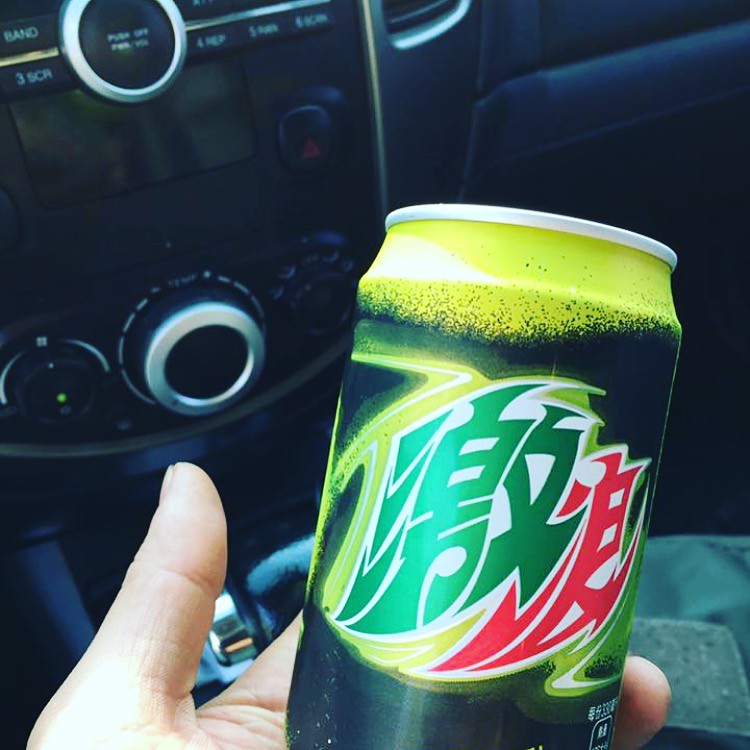In this detailed photograph, a person with a fair-skinned hand holds up a bright, neon green soda can, reminiscent of Mountain Dew’s color scheme, but adorned with green and red Asian script on a white background. The can has a gradation from vibrant neon green at the top to a deep, almost black green at the bottom. The photo is taken inside a car, with the can positioned above the person's green clothing. The car's interior is visibly black, featuring a glove compartment, a radio with silver-trimmed dials, and controls for the air conditioning and hazard button. The thumb, fingers, and a portion of the person's palm are in clear view, showcasing the hand holding the can against the dashboard and the vent to the right.